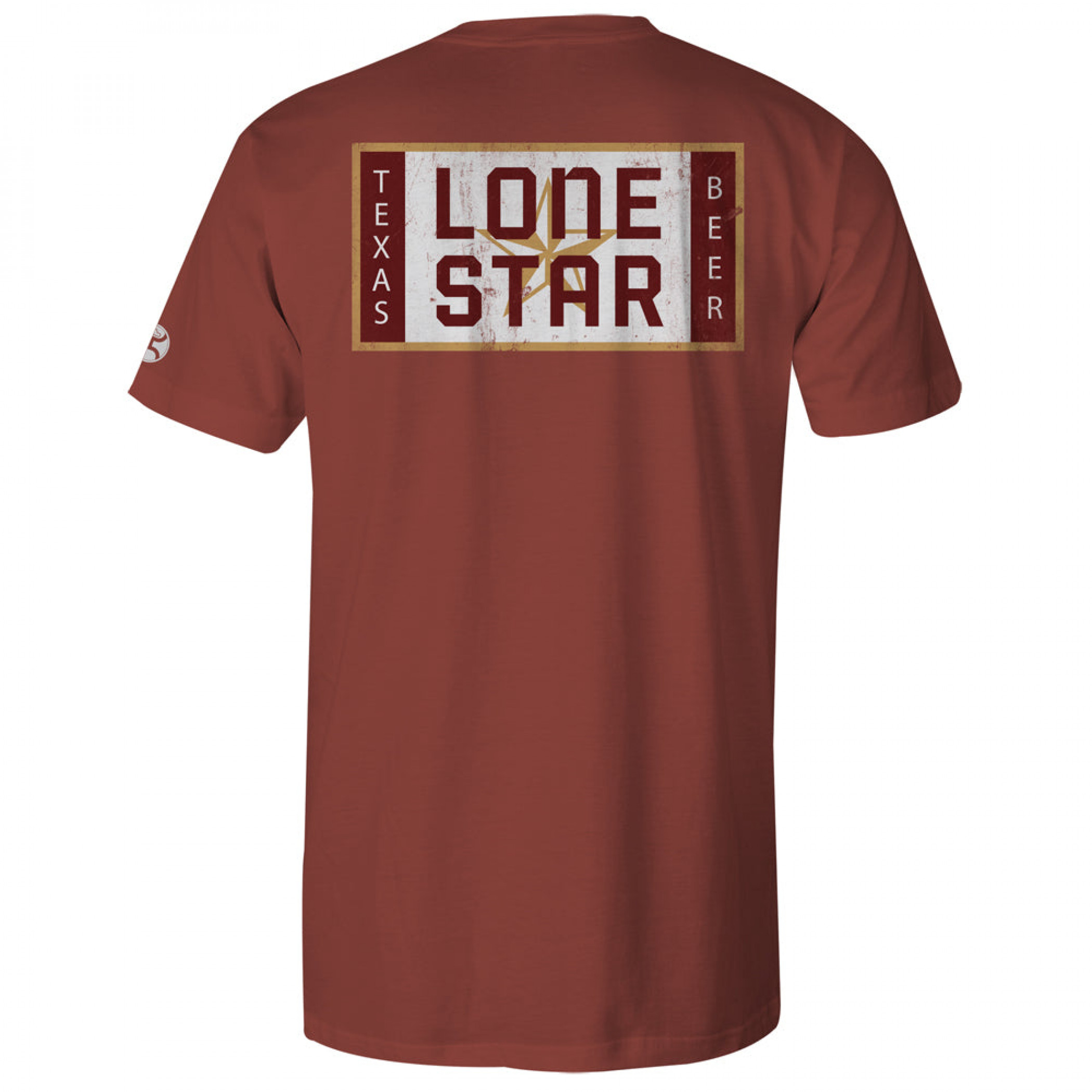This image shows the back of a men's short-sleeved, crew-neck t-shirt in a burgundy red color. The t-shirt appears against a solid white background. Prominently centered on the upper back portion is a rectangular design. This rectangular box is outlined in a gold color. Inside the box, on the left side vertically, it says "Texas" in white font, and on the right side vertically, it says "Beer" also in white font. In the center of the rectangle is a yellow background with the words "Lone Star" in burgundy red font. Below "Lone Star," there is a gold and white five-pointed star that is embossed. The image suggests the presence of a white oblong logo or marking on the left sleeve, just above the hem, though it is partially cut off in the view. The overall aesthetic blends the deep, reddish brick color of the shirt with the contrasting colors and designs of the logo, emphasizing its connection to "Texas Lone Star Beer."